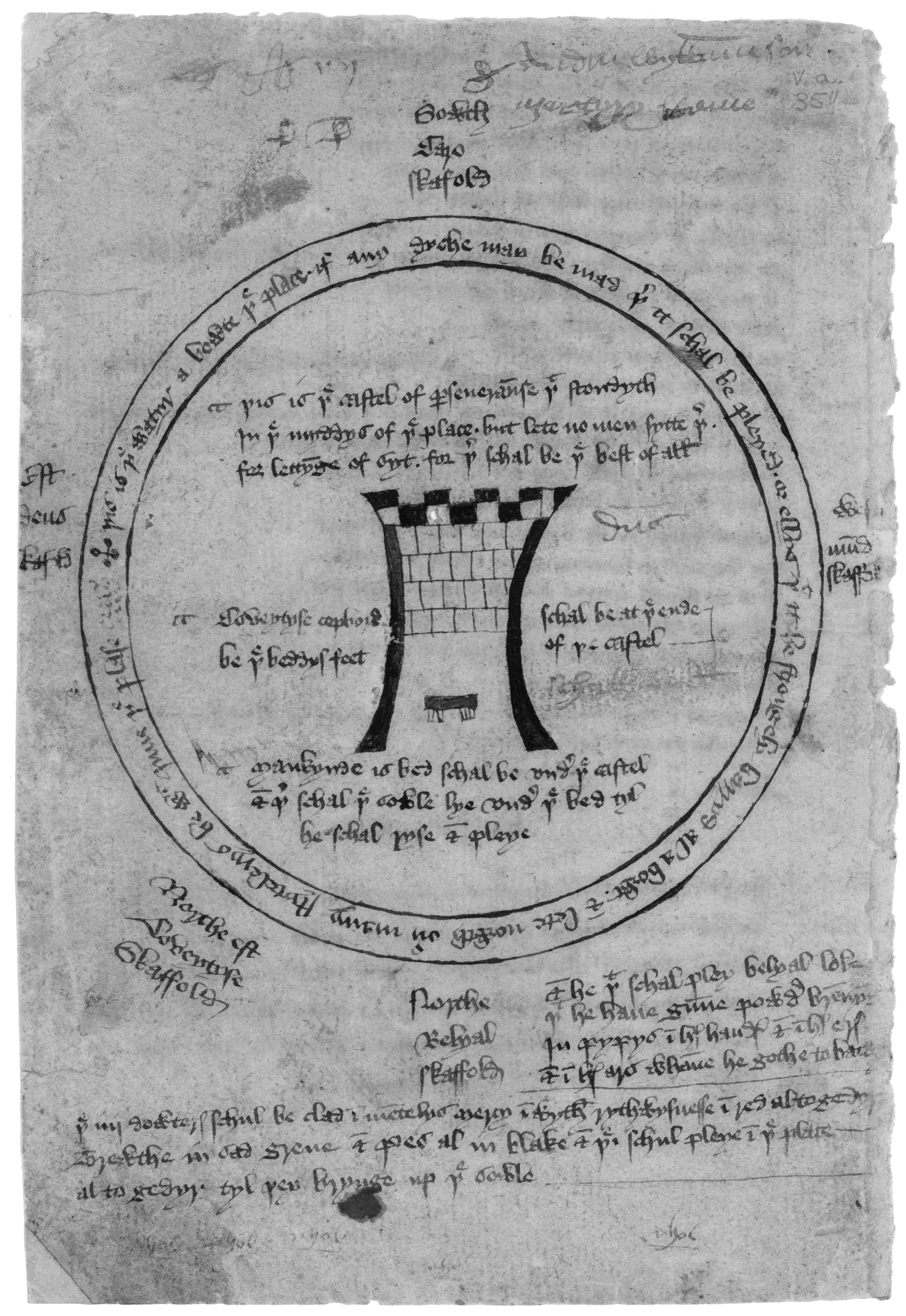The image depicts a worn, gray page appearing as though it was torn from a book due to its jagged right edge. The page is slightly smudged and has an aged, oxidized appearance. At the center of the page is a black circle with an outer layer of text written in an unknown script, resembling either Arabic or Hebrew. Surrounding the circle are sections of fine handwriting that mirror the style found in Medieval manuscripts. Inside the circle, there is an illustration of a structure resembling a medieval castle wall, with a black and gray checkered top, evoking the look of goalposts with a roof. The drawing and text convey a mystical or archaic atmosphere, reminiscent of a pagan ritual or spell.